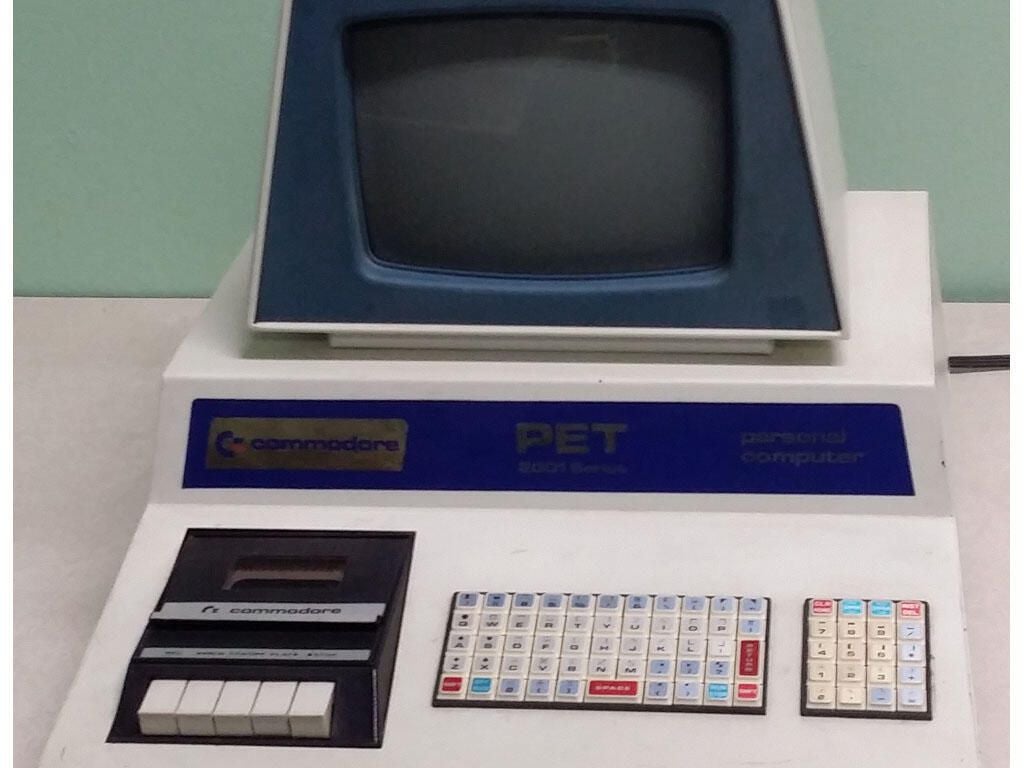This close-up image showcases a vintage Commodore PET personal computer, distinguished by its white base and compact design. The centerpiece is a tiny black screen encased within a blue front and a white plastic frame, with a rounded, almost hexagonal shape. Below the screen, a blue banner prominently displays the Commodore logo in silver on the left, the word "PET" in silver in the center, and "Personal Computer" on the right. The small keyboard area features a very tiny rectangular keyboard with a diverse color scheme: the space bar is red, surrounded by baby blue and white keys, while the arrow keys and some function keys are blue. To the right of the keyboard is a separate, small, square-shaped numeric keypad. On the far left, a black tape deck with five white buttons completes the setup. The image background includes a light gray, triangle-shaped bottom left corner and a mint green square that suggests the room's wall, while the overall close-up perspective emphasizes the computer, making it the focal point of the photograph.